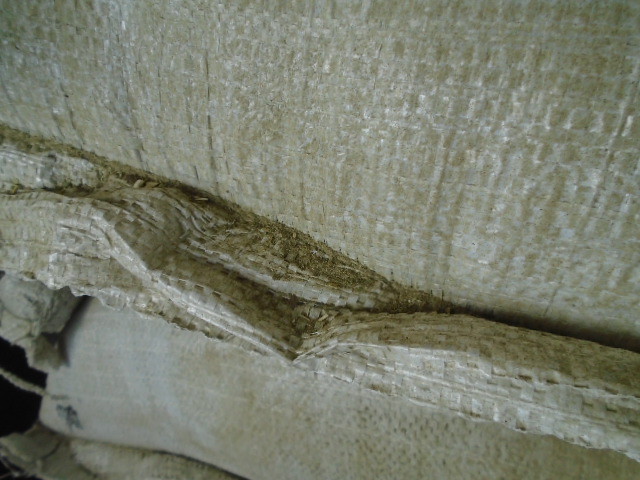The image is a color photograph in landscape orientation, capturing a section of fabric that is likely part of a piece of furniture or a curtain. The fabric, resembling a beige-colored tweed, is predominantly smooth and slightly shiny at the top, woven in nature. Running horizontally across the middle is a crumpled segment where the fabric gathers and folds, protruding from the main surface. Several loose strings hang from this area, adding texture to the composition. Particularly noticeable is a long string dangling from the bottom left corner, accompanied by a black mark. The overall design gives a sense of realism and texture, with the left top portion being narrower and the right side more expansive. Below the gathered fabric are two more items, possibly pillows or fabric extensions in a similar beige hue, further enriching the scene's texture and depth.